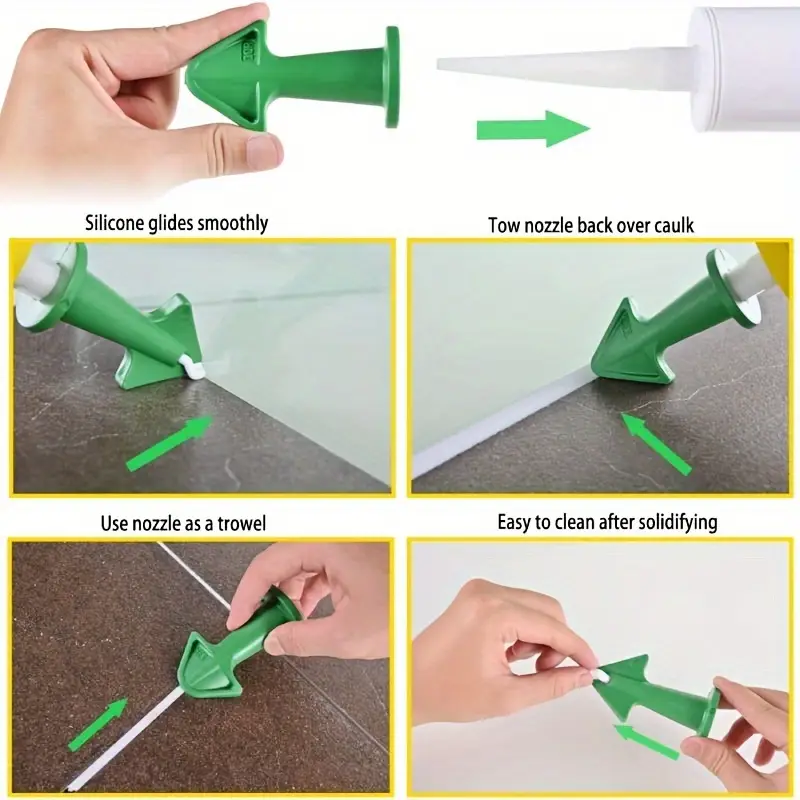The image depicts a detailed set of instructions for using a silicone pump. At the top, a hand holds a green, triangular-shaped nozzle next to a white, pointed cap corresponding to a cylindrical caulking tube. An arrow indicates that you should connect the green nozzle to the white cap. Below this, there are five photos illustrating the steps: 

1. The first image shows the hand holding the green nozzle with text stating "Silicone glides smoothly," indicating silicone dispensing from the nozzle.
2. The second image advises to "toe nozzle back over caulk," showing the action of smoothing the caulk.
3. Additional steps include using the nozzle as a trowel for precise application.
4. The final images highlight the ease of cleaning the nozzle after the silicone solidifies, depicting a person removing the solidified silicone from the nozzle.

These comprehensive instructions make the process of assembling, using, and cleaning the silicone pump straightforward.